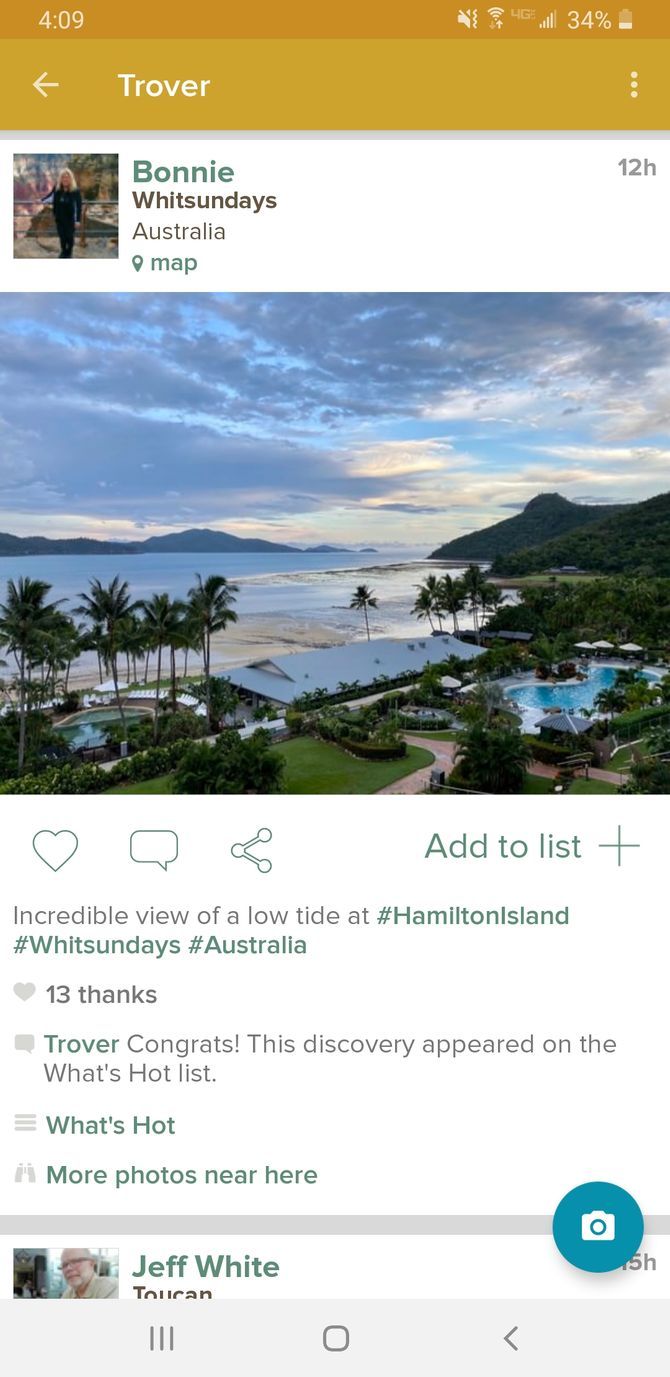This image is a screenshot displaying a photo-sharing application interface on a mobile device. At the top of the image, there's an orange-brown border showing the time as 4:09 and a battery icon indicating 34% remaining. Below the border, a tan banner with the word "Trover" written in white is visible.

Directly underneath the banner, there's a white area containing a user profile section. This section features a rectangular image of a woman in front of some rocks, labeled "Bonnie" in green text. To the right of Bonnie's name, it says "Whitsundays, Australia," accompanied by an icon of a map and the time "12H" ago.

The main content of the screenshot is a large image showcasing a scenic resort. The scene includes a vibrant blue sky with scattered clouds, an ocean view on the right, and several palm trees lining the beach. In the foreground, there is a swimming pool surrounded by patches of grass. The caption on this image reads: "Incredible view of a low tide at #HamiltonIsland #Whitsundays #Australia," followed by "13 thanks." A response from Trover congratulates the user, noting that the discovery appeared on the "what's hot" list and suggests that there are more photos from this location.

Additionally, the interface at the bottom hints at further exploration with the prompt "what's hot, more photos near here."